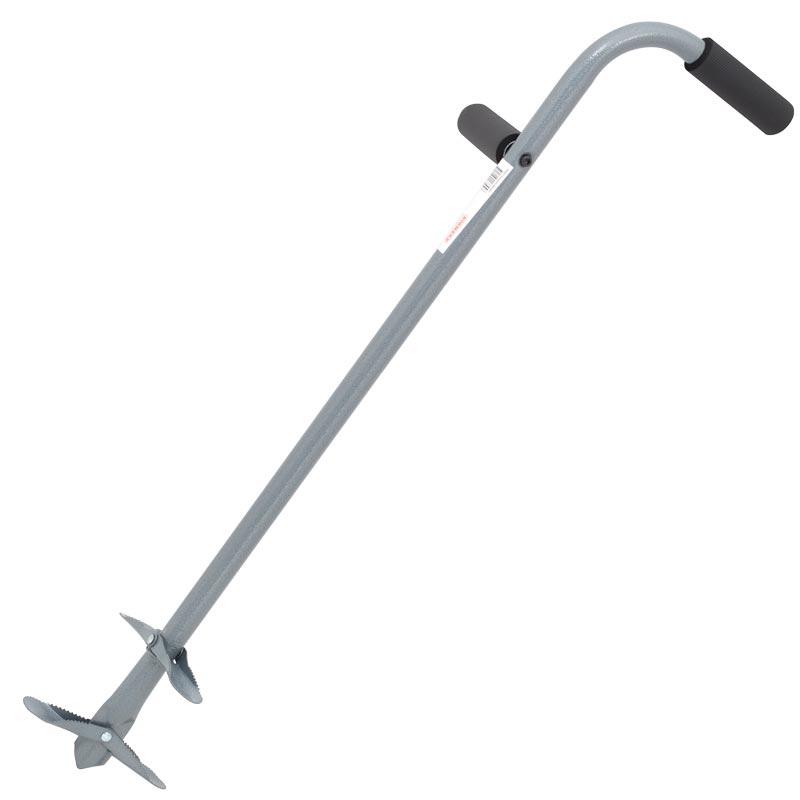This image displays a unique, dark gray metal tool with a shiny finish, reminiscent of a cane but likely an agricultural implement like a hand tiller or soil aerator. The vertical main shaft features two handles: one at the top, curving and equipped with a black grip for comfortable holding, and another perpendicular handle a few inches below, fixed in place with a visible black screw. A white label with a barcode is attached beneath the top handle. The tool bottom transitions from a rounded pole to a flattening that splits into two metal extensions with serrated, toothed edges, resembling small grasping prongs or blades. These prongs are hinged, suggesting they can move or rotate, possibly to penetrate or twist soil for aeration. The background is a plain white, emphasizing the detailed construction of the implement.